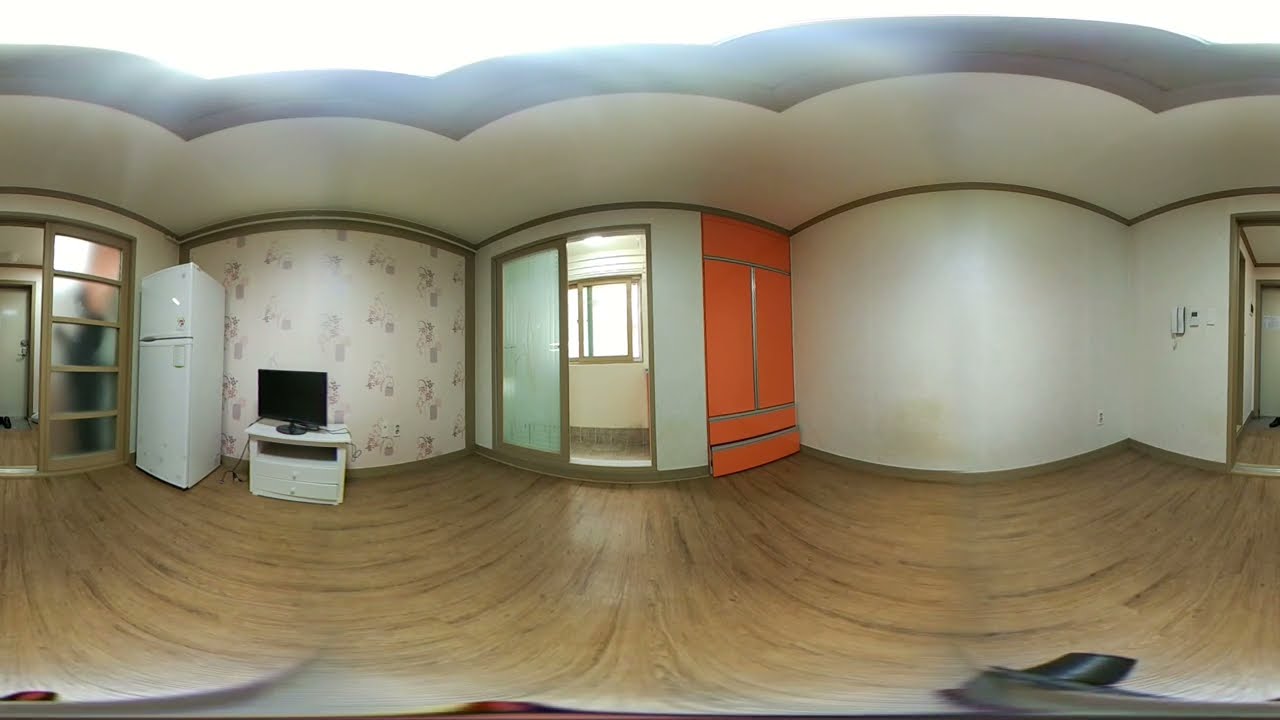The image provides a detailed view of a sparsely furnished living room, likely captured with a fisheye lens giving a 360-degree perspective. Dominating the left side of the room is a white, single-door refrigerator with a top freezer. Adjacent to it is a small, white table acting as a TV stand, featuring two drawers below and a compact, black flat-screen TV or computer monitor, positioned as if unplugged. The backdrop of this section shows an intricate floral wallpaper in light pink, while the surrounding walls are primarily white. 

The right side reveals an entrance leading into a hallway and an orange wall featuring a built-in cabinet with a silver trim. Further to the right, a mirrored closet door stands alongside a section of frosted glass, through which the silhouette of a person can be discerned. The wooden floor, in a blend of white and brown hues, extends across the room. The ceiling remains white, maintaining a minimalistic and somewhat transitional ambiance, suggestive of someone either moving in or out of the apartment.